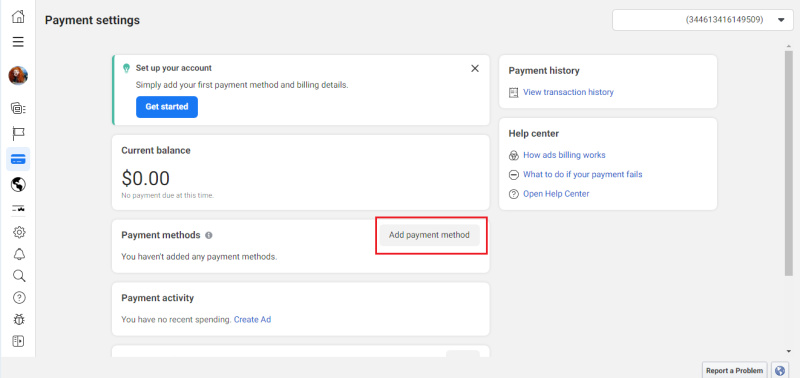This image depicts the payment settings interface of an account setup screen. The user is prompted to add their first payment method along with billing details to get started. The current account balance is displayed as $0.00, with no payments due at present. The "Payment Methods" section indicates that no payment methods have been added yet, and includes an option to "Add Payment Method." The "Payment Activity" section shows no recent spending, and there's an option to "Create Ad." Under "Payment History," users can view their transaction history.

Additional resources are available, including a "Help Center" with links explaining how ad billing works and instructions on what to do if a payment fails. Users can open the help center or report a problem directly from the interface.

A distinctive feature at the top right corner of the screen is the identification number: 344-6134-161-49509. In the bottom right corner, there is a "Report a Problem" option.